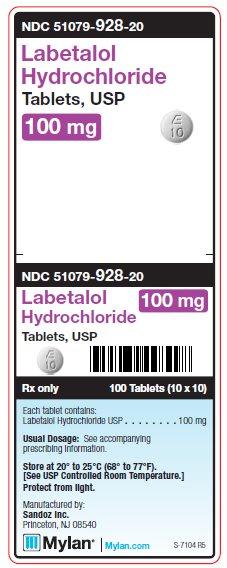The image displays a white box with a pinkish-purple border. At the top of the box, "NDC 51079-928-20" is printed. Below this, in purple text, "Labetalol Hydrochloride" is stated, followed by "Tablets USP" in black text. Another purple box within the design indicates "100 mg." Additionally, a detailed illustration shows a round pill with a unique design above it. 

Further down, the previously mentioned NDC number, "NDC 51079-928-20," is reiterated. The description "Labetalol Hydrochloride 100 mg Tablets USP" appears again, accompanied by another image of the pill. On the right side of the box, a barcode is displayed, and underneath it, the text "RX only, 100 tablets (10 x 10)" is printed. 

Beneath these details, a blue tab is present, stating: "Each tablet contains Labetalol Hydrochloride USP, 100 mg. The usual dosage is specified in the accompanying prescribing information. Store at 20°C to 25°C (68°F to 77°F)."